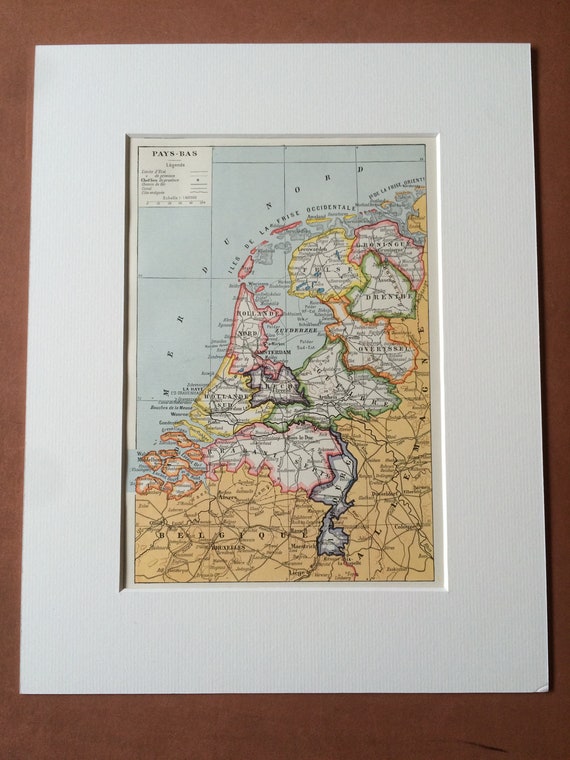This image captures a detailed, realistically depicted map mounted on a dark brown wall, encased within a gray border. The map, seemingly not in English, portrays a coastal region, potentially Northern Europe, featuring the topographical complexity of an ocean labeled "MER DU NORD" in the top left corner. Outlined in vibrant colors such as pink, yellow, green, orange, and black, various sectors within the map indicate different regions or sovereign entities. The interior regions of these outlines typically appear white, with additional shades of blue and dark blue accentuating other areas. A conspicuous bay intrudes into the landmass, further enhancing the coastal detail. The bottom section of the map contains intricate black lines that likely represent roads or geographical features, all supplemented with hard-to-read black text. The map’s meticulous division into quadrants and the presence of a box labeled with incomprehensible text in the corner add to its intricate and scholarly presentation.